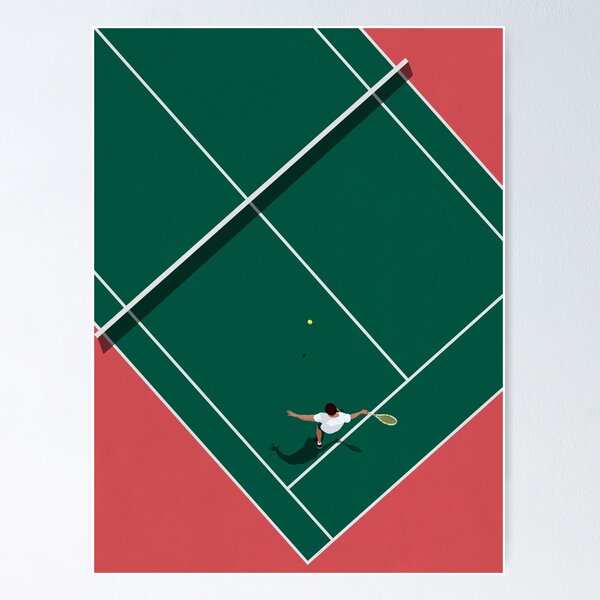This image is a created, perhaps digitally generated, aerial view of a vividly detailed tennis court scene. The background is primarily a soft grey or white, with the central figure being a diagonal depiction of a green tennis court bordered by reddish-pink triangles in each corner. The court features white markers and a white diagonal line representing the net, though the net's mesh isn't visible. Positioned in the lower left quadrant of the court, a lone player with black hair is poised to hit a yellow tennis ball. He wears a white t-shirt, blue shorts, white socks, and black athletic shoes. His right hand grips a yellow racket, and his arm is drawn back in mid-swing, shadow below indicating the ball is suspended mid-air. The entire scene is framed by a thin white border, completing the composition of this meticulously illustrated tennis-themed art print.